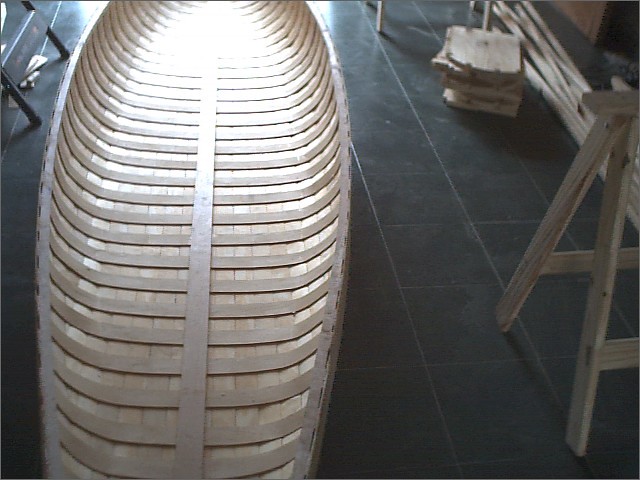In an indoor workshop, likely a garage, the image captures a beautifully handcrafted wooden longboat or canoe, still under construction. The canoe, resembling the shape of a kayak, and constructed with a series of meticulously bent, blonde wood pieces, sits on a dark gray, tiled floor. Various structural elements, such as cross pieces, the centerpiece, sides, and rails, are clearly visible, emphasizing its simple yet steady design. Surrounding the canoe, the workshop is scattered with woodworking tools, a metal stool, and stepping stools, alongside a wooden sawhorse on the right. In the background, there is a mix of random plywood pieces and stacks of rough-cut planks and small wood pieces, indicating ongoing woodworking projects and adding to the creative clutter of the space.